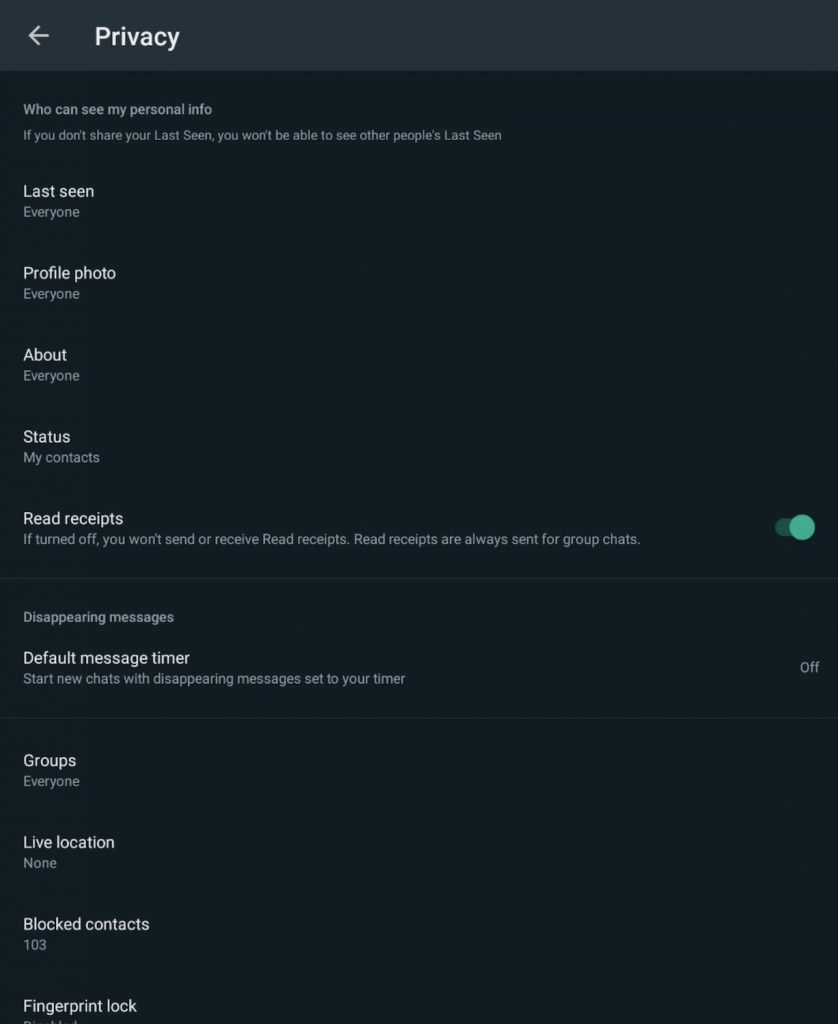The image displays a settings screen from a website in dark mode, featuring a dark navy-colored background with a gray border at the top. At the upper left corner, a white back arrow points left, accompanied by the title "Privacy." Beneath this heading, several privacy settings are detailed as follows:

- **Who Can See My Personal Information**:
  - Last seen: Everyone (Note: If you don't share your last seen, you won't be able to see others')
  - Profile photo: Everyone
  - About: Everyone
  - Status: My contacts

- **Read Receipts**: Active (Green toggle indicating the service is on; Read receipts are always sent for group chats)
- **Disappearing Messages**:
  - Default message timer: Off (Start new chats with disappearing messages set to your timer)
- **Groups**: Everyone
- **Live Location**: None
- **Blocked Contacts**: 103
- **Fingerprint Lock**: The full description is cut off in the image.

This comprehensive setup reflects the user's privacy preferences and controls over their account activity and visibility.